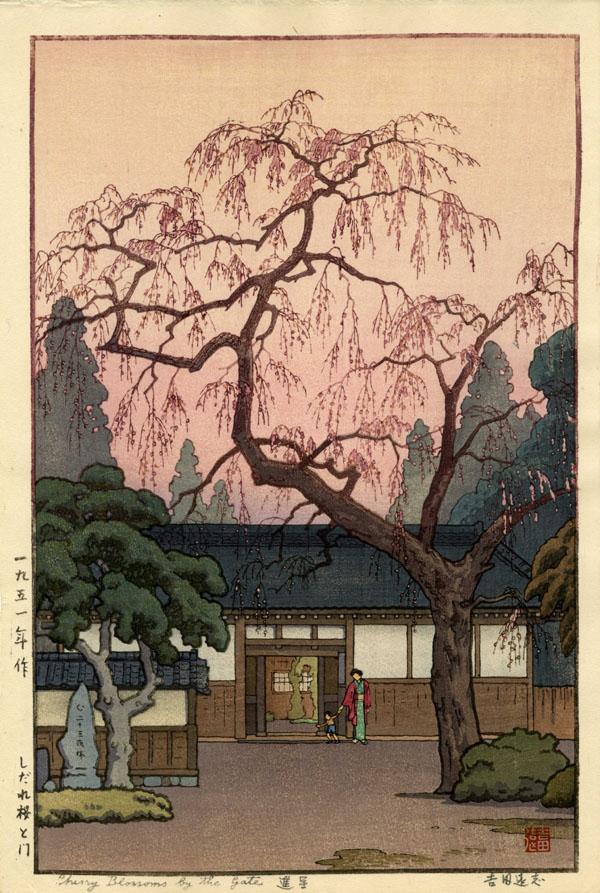This vibrant watercolor painting, reminiscent of a traditional Japanese art print, portrays an idyllic scene characterized by the delicate beauty of a cherry blossom tree. The tree, with its pink blossoms juxtaposed against the similarly toned sky, stands prominently on the right side of the piece. The vertiginous trunk is a rich brown, and it’s flanked by green shrubs rooted in the brown earth.

To the left, a smaller tree with a gray trunk stands beside a gray statue, adding variety to the floral scene. In the background, a pagoda-style building stretches across the middle of the painting, introducing architectural elements into the natural setting. At the base of this building, an Asian woman dressed in a red shirt and green dress walks hand in hand with a small child, suggesting a familial and serene daily life.

Japanese characters elegantly frame the scene, with inscriptions adorning the left side and bottom of the white-bordered painting. These inscriptions include a Japanese stamp signature in the bottom right corner and text indicating the title as "Cherry Blossoms by the Gate." The painting is dominated by hues of pink, red, green, beige, and shades of brown, capturing the quintessence of cherry blossom season in Japan.